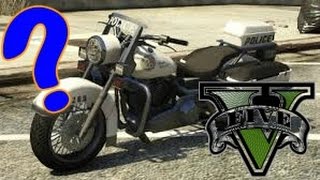This image depicts an old-fashioned white police motorcycle parked on a street, with a light gray sidewalk visible in the background. The motorcycle features a large round headlight encased in a black ring, with a clear lens and a silver handlebar that includes black grips. Prominently displayed on the white front fender is the number "263" in black. The front windshield of the motorcycle, which is small and made of glass, displays the word "POLICE" in white letters. Additionally, the white container mounted on the black seat also reads "POLICE" in black lettering. The motorcycle’s tires have new-looking, deep treads. The front tire is near a large blue question mark with an orange outline located at the top left of the image. At the very bottom right of the image, there is a green "V" partially covered by a clear banner with the number "5" in black letters. The motorcycle is parked on asphalt, over white parking space lines, but not aligned properly within the space. The background reveals the edge of a dark, possibly garbage-filled bag at the top right corner of the image.